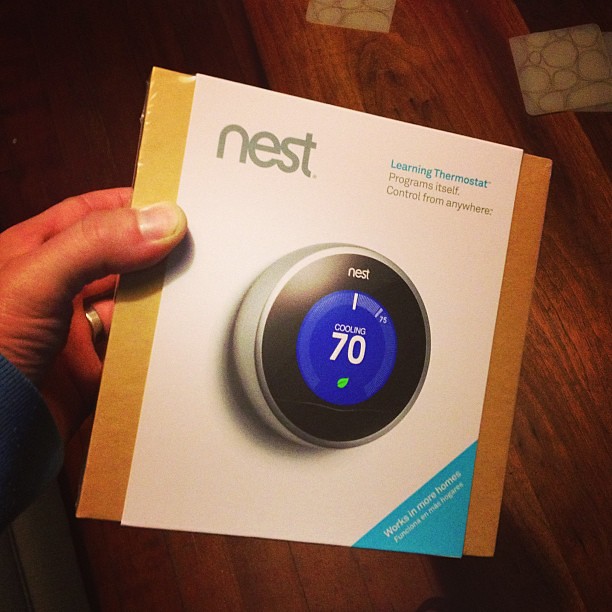In this detailed photograph, we observe a person's hand holding a product box, with the thumb prominently positioned on top of the box. The front face of the box is primarily white, complemented by a yellow background. Grey letters spell out "N-E-S-T" on the main white section. To the right, blue text states, "learning thermostat," followed by "programs itself" and "control from anywhere." The center of the box features a circular thermostat, clearly labeled "nest" with a blue circle in the middle. Digitally displayed within the circle, the word "cooling" and the number "70" appear in white, accompanied by a small green leaf icon underneath. In the lower right corner of the box, a blue section announces, "works in most homes." 

The background of the image reveals a wooden surface, which could either be a floor or a table. In the upper right corner of the photograph, there are two light grey squares, each adorned with images resembling circles or stones.